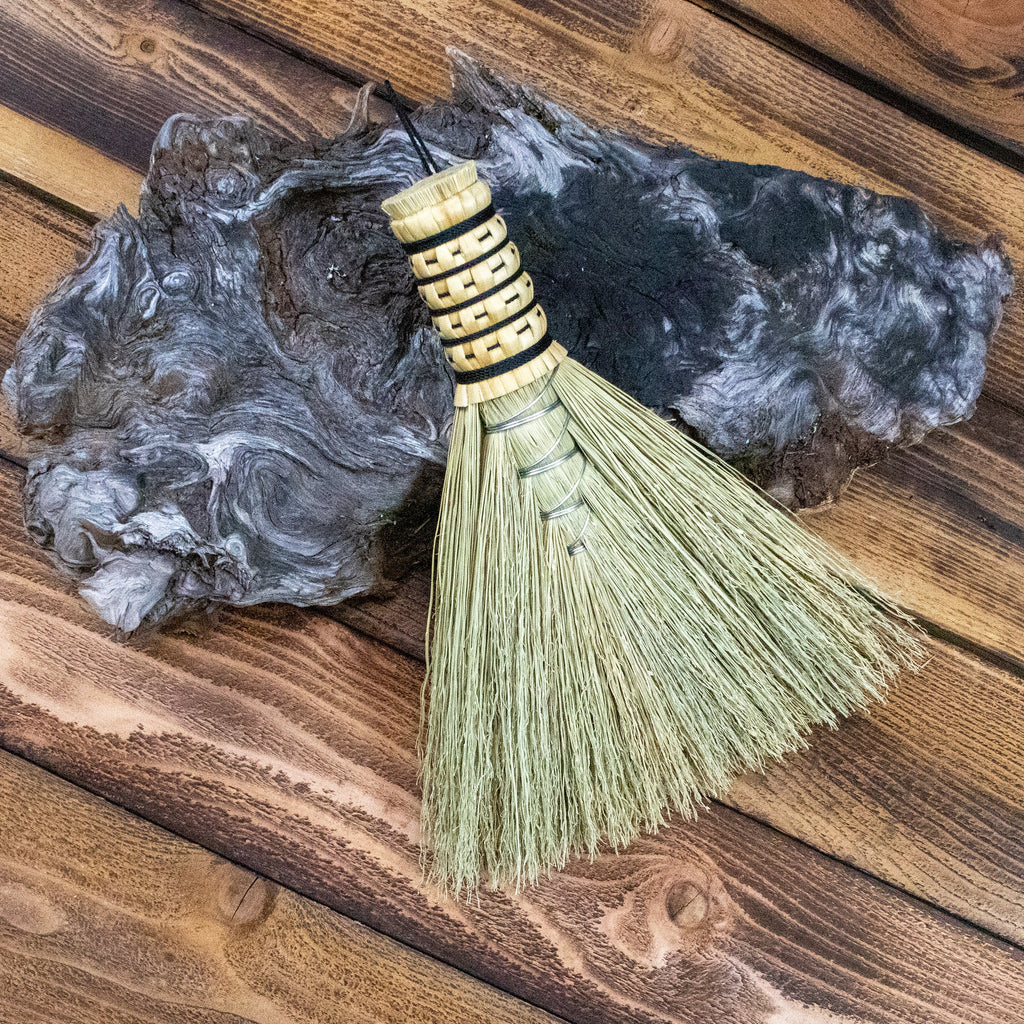In the image, a small, triangular-shaped straw broom with a short wicker handle wrapped in black horizontally is lying atop an old, weathered, oval-shaped piece of wood. This slab of wood has a grayish-black and white swirly pattern resembling ink dropped in water and stirred around, with areas that are starkly black. The broom’s bristles fan out in a triangular shape and are a tannish-green color. This setup rests on a medium-toned wooden floor (or possibly a tabletop) with visible knots and lines in the slats, arranged diagonally from left to right. The image is taken from an above-angle shot, with the broom positioned so that its handle points upwards and its bristles point towards the bottom right. The overall color palette includes various shades of dark gray, off-white, tan, yellow, dark brown, and light brown. The background wood grain and the worn texture of the slab create a rustic atmosphere focused on the broom as the central subject.